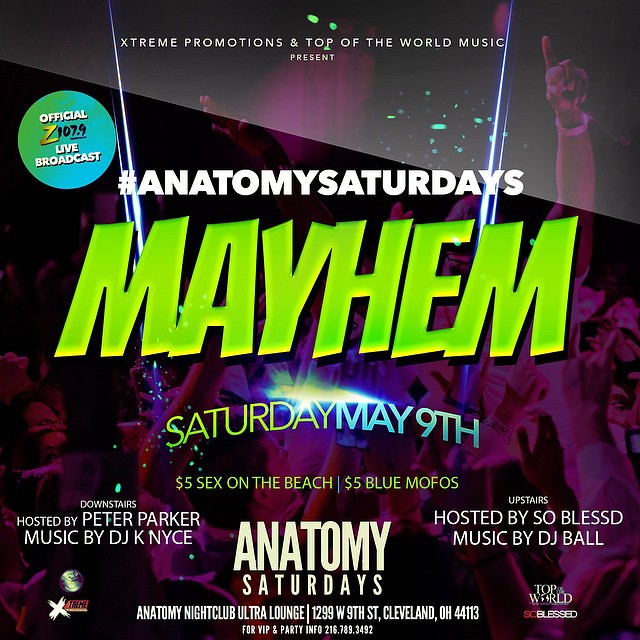The promotional image is a tall rectangular poster for a nightclub event with a dark, party-themed background showcasing a crowd of people with their hands up, captured in purple and red hues. In the center of the image, eye-catching, large neon green text with a yellow tint boldly announces "MAYHEM." Just above this, in thick white, all-capital letters, it reads "HASHTAG ANATOMY SATURDAYS." At the very top, in smaller white, all-capital letters, it states "EXTREME PROMOTIONS AND TOP OF THE WORLD MUSIC PRESENT."

Below the word "Mayhem," in text that transitions from neon green to bright blue, it reads "Saturday May 9th." Following this, in green font, all capital letters, it advertises "$5 Sex on the Beach, $5 Blue Mofos." Towards the bottom left corner, in smaller white text, it mentions "Downstairs hosted by Peter Parker, music by DJ K Nice," while the far right corner indicates it is "Hosted by Blessed, music by DJ Ball." Additionally, there is a blue and green circular logo near the top left labeled "Official Z 107.9 Live Broadcast." 

Overall, this vivid and detailed poster promotes a vibrant nightclub event filled with live music, special hosts, and enticing drink offers.